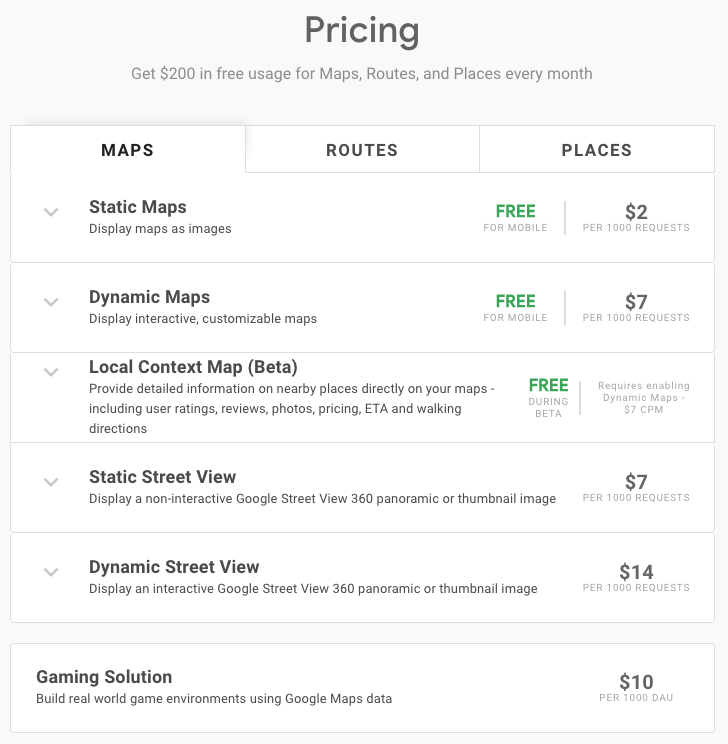In this detailed image, we observe a screenshot set against a light gray background. At the top, the word "Pricing" is prominently displayed in bold black text. Directly below, in light gray text, the message "Get $200 in free usage for maps, routes, and places every month" is stated.

The interface features three white button tabs that are arranged horizontally from left to right, each labeled in bold black text: "Maps," "Routes," and "Places." Underneath these tabs, there's a section titled "Static Maps," marked by a pull-down arrow on the left. Directly beneath this title, "Display maps as images" is written in smaller text. To the right, "Free for mobile" is highlighted in green text, and beside it, " $2 per 1,000 requests" is noted in black text. 

Following this section, another line reads "Dynamic Maps" in bold black text, accompanied by another pull-down arrow on the left. Below this heading, in light gray text, it says "Display interactive customizable maps." Similarly, to the right, "Free for mobile" is again indicated in green text, with "$7 per 1,000 requests" written in black text nearby.